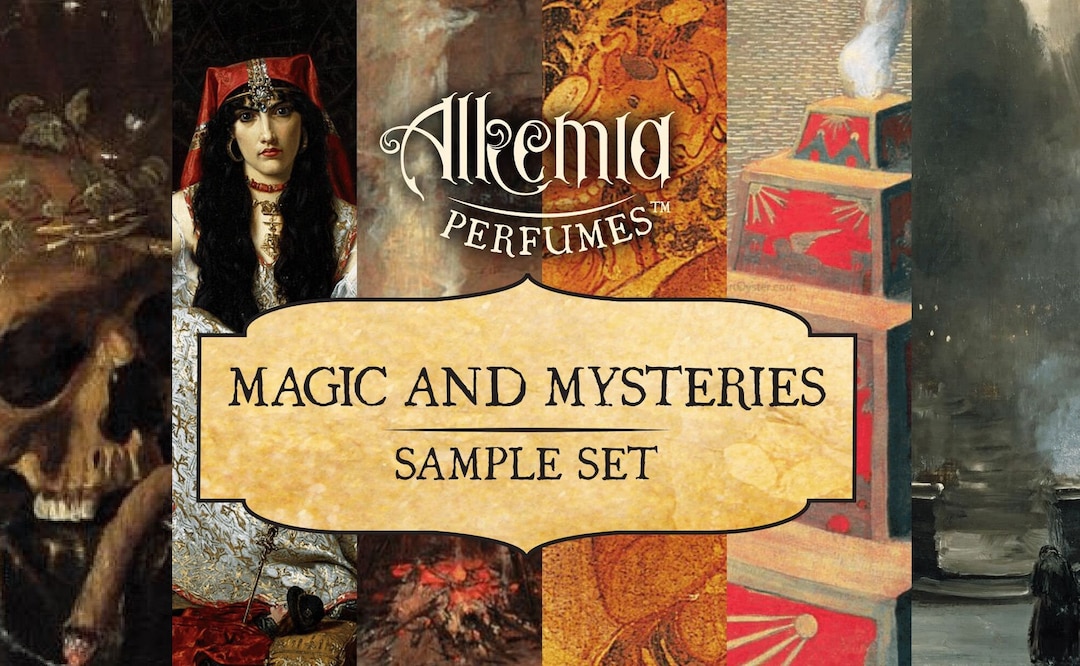The image is a detailed advertisement or label for the "Alchemia Perfumes Magic and Mysteries Sample Set." The type setting used gives it a mystical, witchy feel, suitable for attracting witches and warlocks. The text "Alchemia Perfumes" is prominently placed at the top, with "Magic and Mysteries Sample Set" below it. Vertically aligned on the left side are six distinct images: 

1. A brown skull adorned with jewels above it.
2. A woman with long black hair, wearing a red headdress and a robe of silver and gold, evoking a pirate or gypsy aesthetic.
3. An abstract, smoky fire-like pattern.
4. A yellow Buddha-like figure surrounded by intricate patterns.
5. A stack of boxes, with smoke wafting from the topmost one.
6. A black and white street scene featuring a car at the bottom, hinting at a nighttime ambiance.

These elements combine to create a striking, evocative visual that captures the essence of the mysterious and enchanting theme of the perfume set.